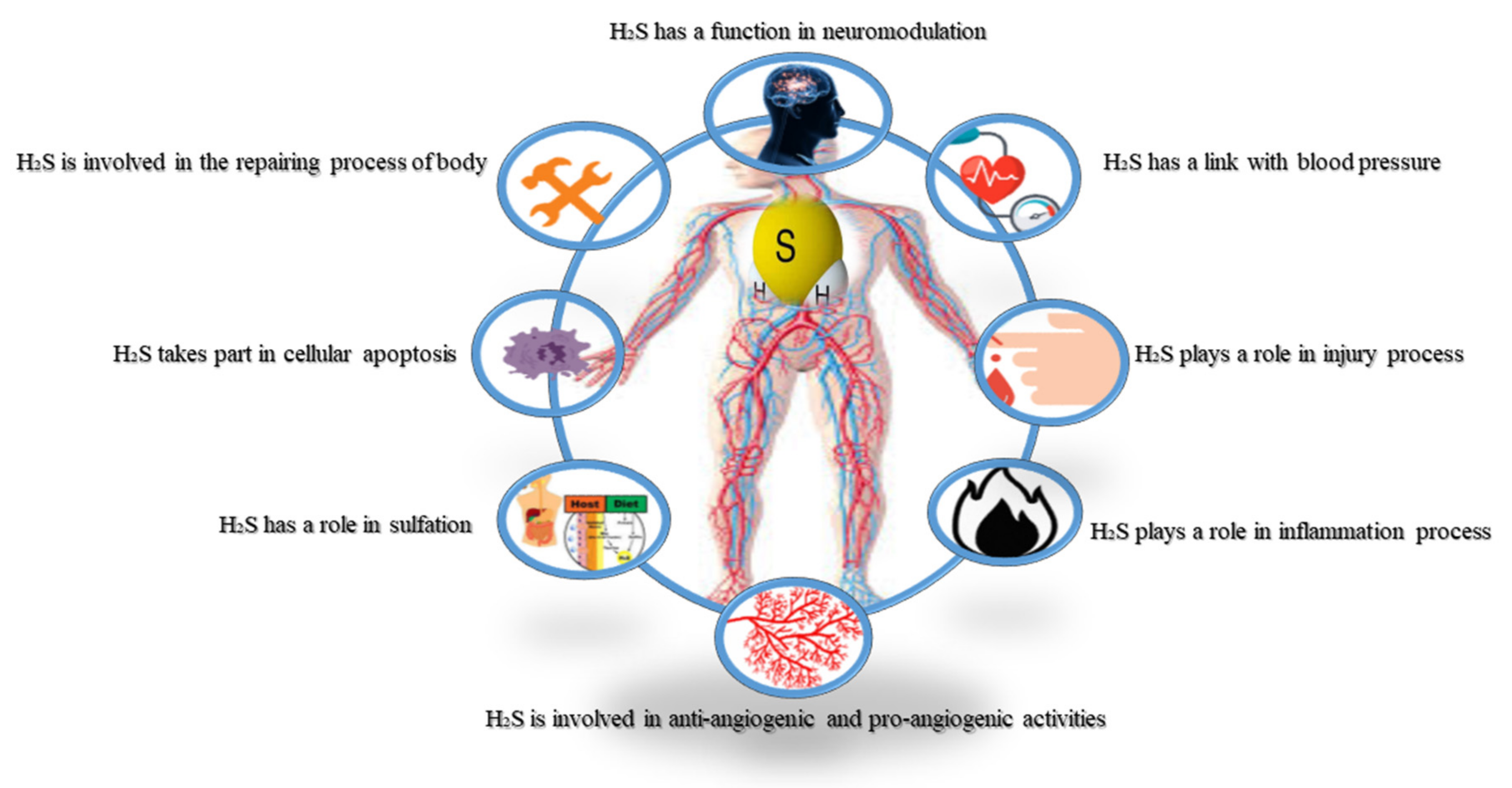This detailed, color illustration, likely from a science or biology textbook, showcases a computer-generated anatomical diagram of a generic human figure with white skin, depicting the entire cardiovascular system in a transparent view. Red and blue-colored veins and arteries stretch from the head to the feet, emphasizing the extensive network of blood vessels. Central to this image is the role of hydrogen sulfide (H2S) in various physiological processes, highlighted by text and symbols arranged in a circular, clockwise fashion around the figure. The text notes that H2S has functions in neuromodulation, is involved in the body's repair processes, has a link with blood pressure regulation, plays a part in cellular apoptosis, and has roles in the injury and inflammation processes. Additionally, H2S is noted for its involvement in both anti-angiogenic and pro-angiogenic activities as well as in sulfation processes. Various symbols, such as a heart, tools, and flames, visually reinforce these functions and conditions related to the human body.